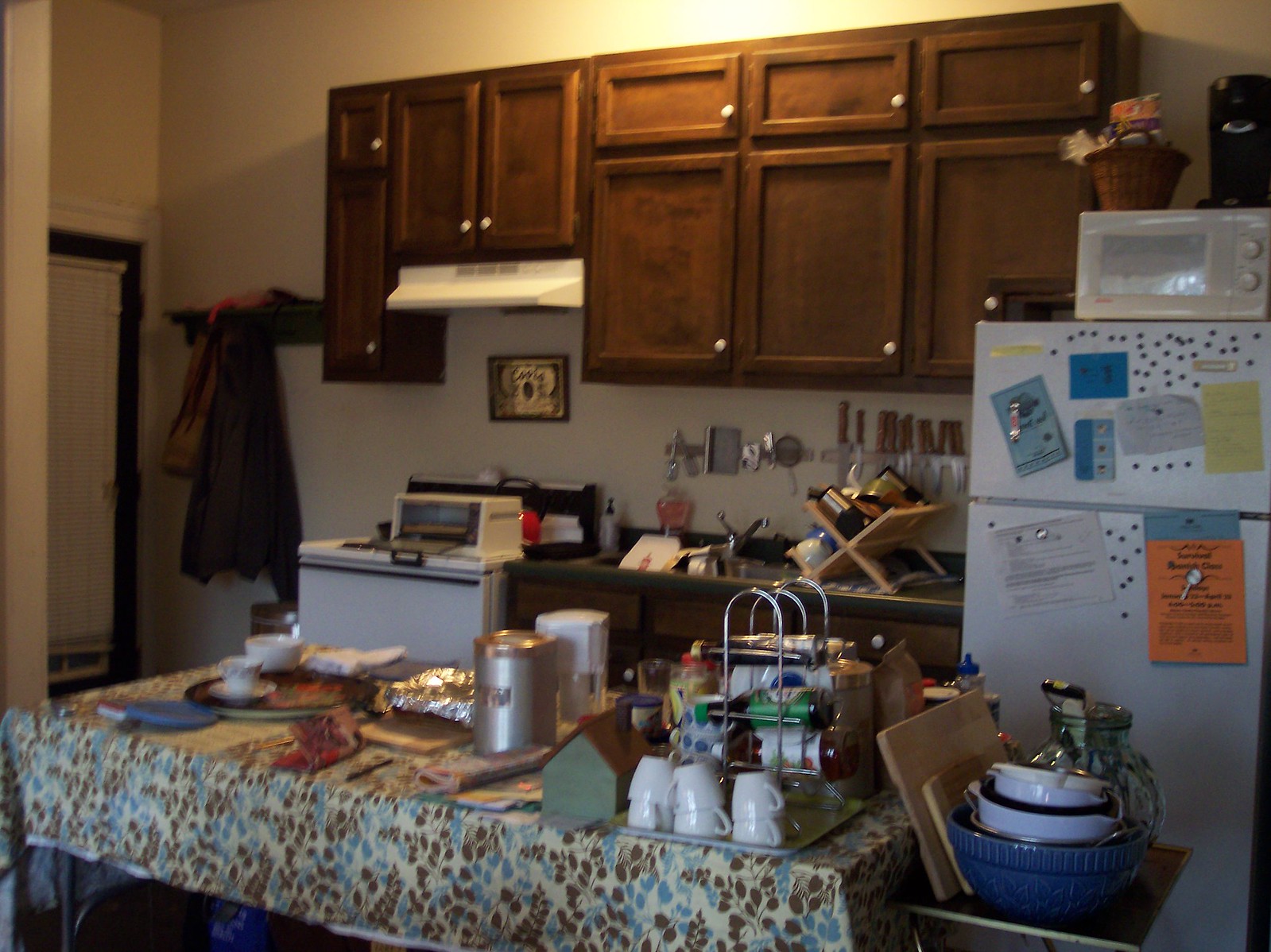The image depicts a bustling, well-organized kitchen that appears to be arranged for a party. At the center of the kitchen stands a dining table, adorned with various dishes and drinkware, suggesting preparations for an upcoming social gathering. Surrounding the table are modern appliances, including a prominent refrigerator with assorted documents and papers affixed to its door, adding a personal touch. The countertops are tidy, with a selection of ingredients and utensils hinting at ongoing culinary activities. The overall atmosphere exudes anticipation and warmth, highlighting the heart of the home ready to welcome guests.